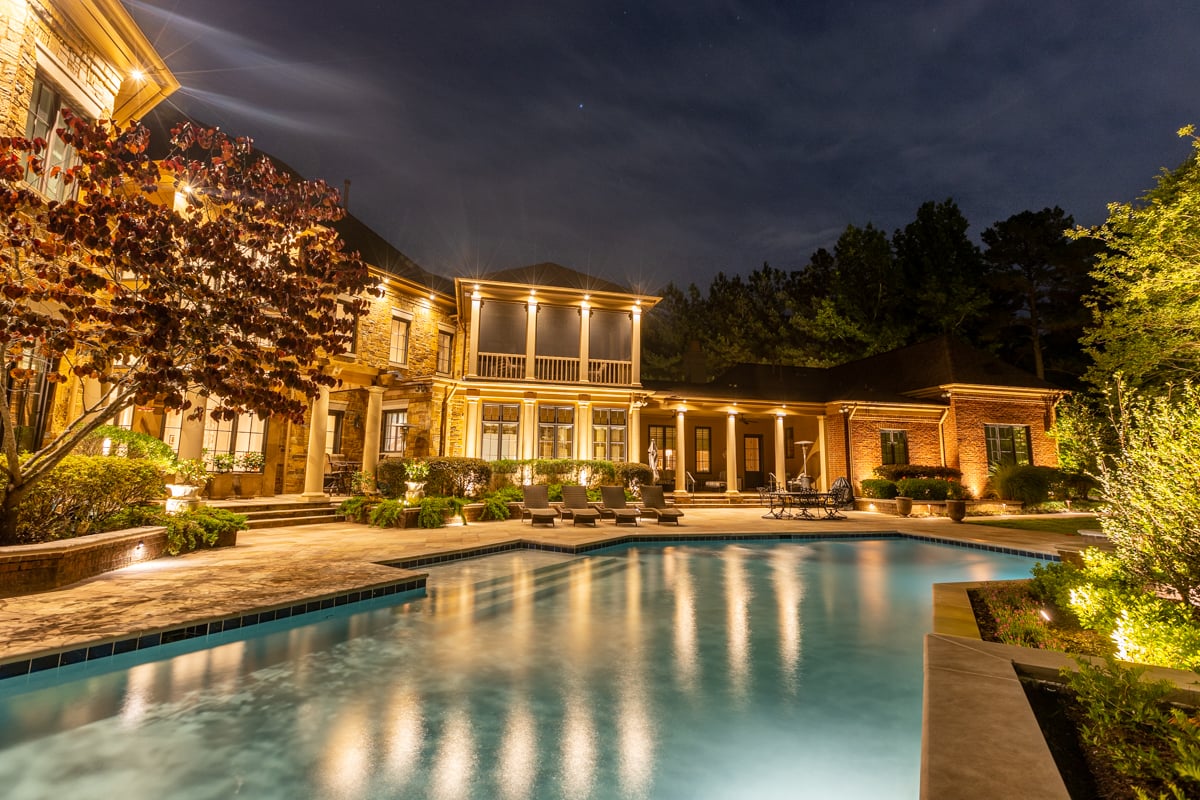This night-time photograph captures a grand mansion, with the main focus on its striking architectural features and expansive outdoor space. The foreground of the image is dominated by an enormous, crystal-clear swimming pool that takes up nearly half of the frame. The mansion itself, illuminated by warm lighting, appears to be built around the pool, creating a cohesive and integrated design.

The mansion boasts a beautiful stone facade that adds a touch of timeless elegance to its appearance. The structure is primarily two stories, although the right side of the building in the foreground is a single story, adding an interesting variation to its silhouette.

Surrounding the pool is meticulously maintained landscaping that includes a variety of shrubbery and strategically placed planters, enhancing the overall aesthetic appeal. Stone stairs lead up to different levels of the garden, while benches invite guests to sit and take in the serene atmosphere. The image perfectly captures the opulence and thoughtful design of this luxurious property.